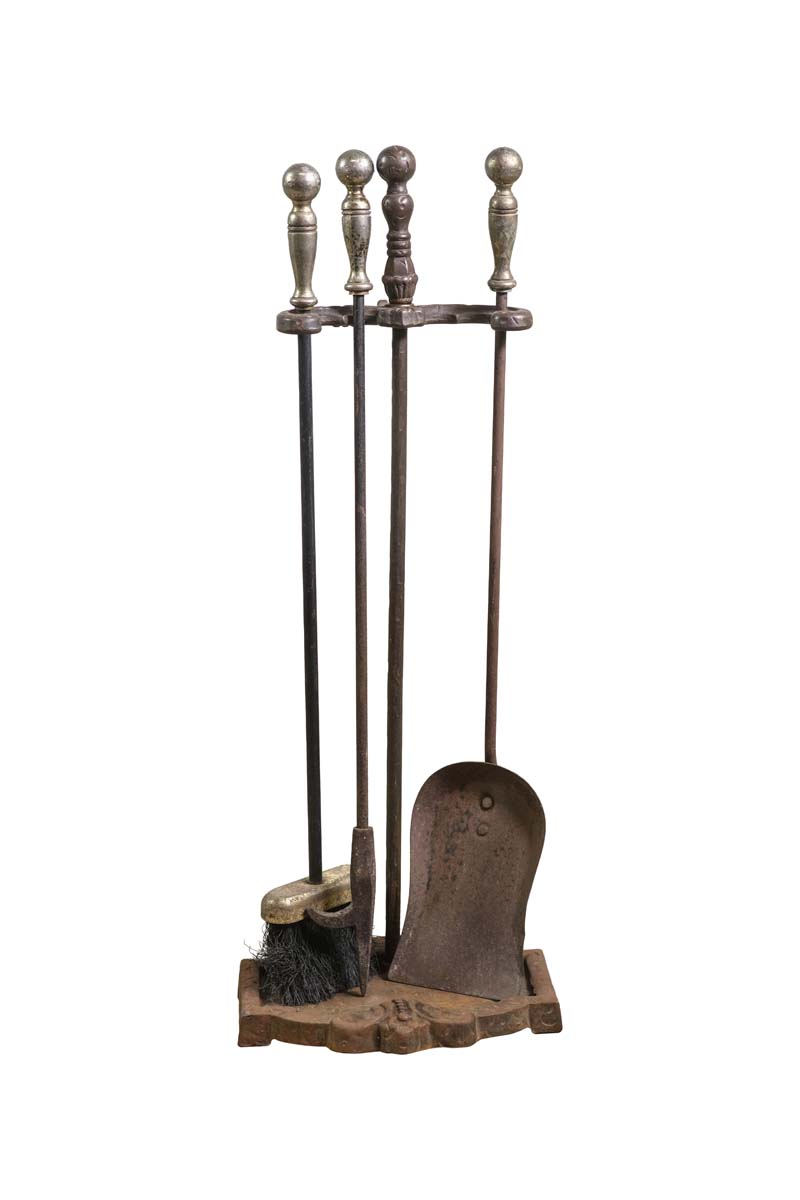The image showcases a set of aged and rusted tools designed for cleaning and tending to a fireplace. The tools, which include a shovel, a fire poker with a spear-shaped tip, a log hook, and a broom with black bristles, are mounted on a tarnished and discolored steel stand. Each tool features a long black shaft with a silver handle topped by a round ball, adding a touch of classic design despite their worn condition. The shovel, prominently rusted, and the dustpan, which also shows signs of significant wear and rust, sit alongside the rusty broom, indicating frequent use. The flat metal base of the stand, adorned with a design at the front center, supports the tools, which rest on hooks at the top of the frame. The entire set exudes an aged charm, reflecting its extensive use in maintaining fireplace hygiene.